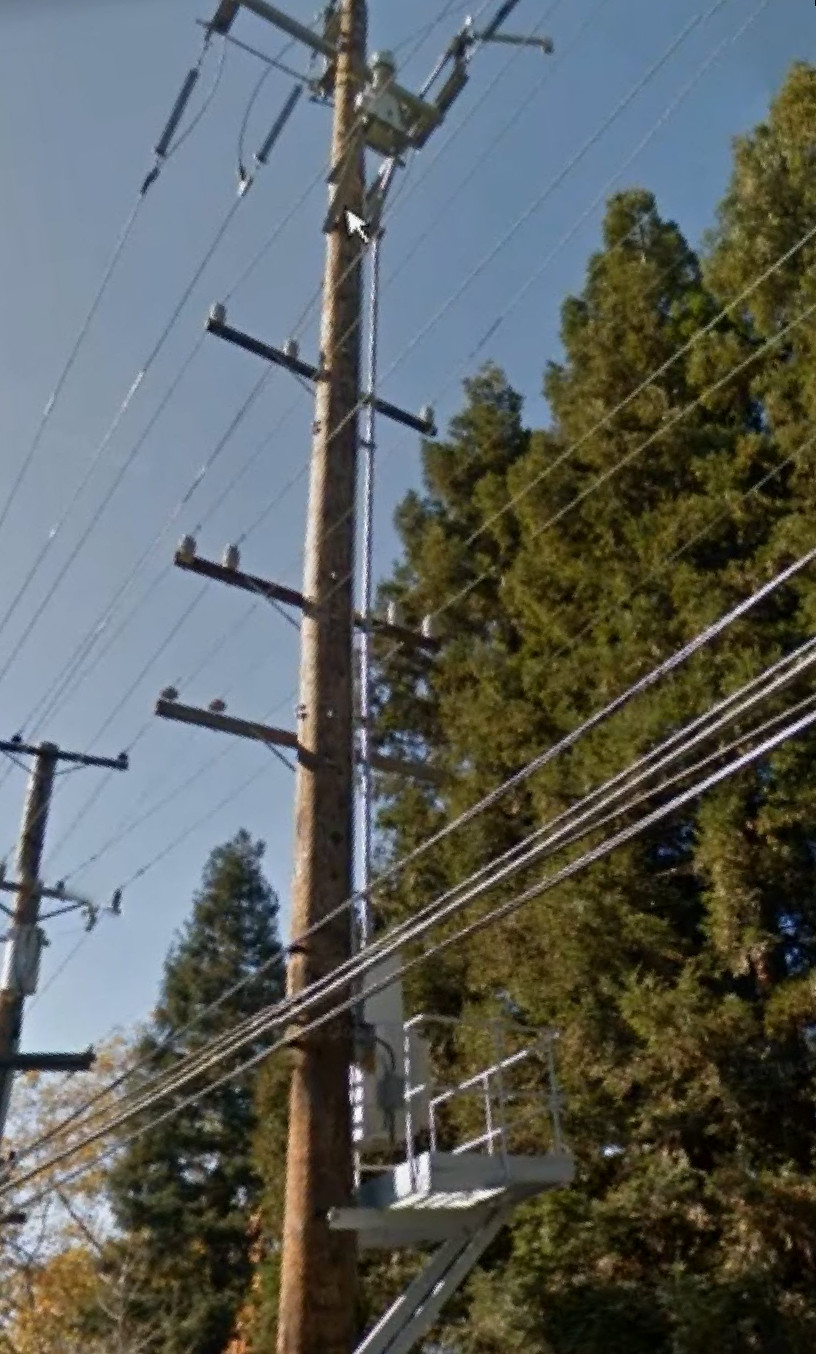In this daytime outdoor image, a tall wooden utility pole dominates the scene, reaching high into a clear medium-blue sky. The pole supports a complex network of heavy-duty electrical wires, mounted with metallic rods, coils, and spring-like machinery. Connected to the pole are multiple dark-colored metal pieces and a dense bundle of wires that are too numerous to easily count. The wires stretch outward, linking this pole to another beyond the frame. Positioned at the base of the pole is a white cherry picker with extended metallic legs and a surrounding cage, indicative of equipment used by line workers for repairs. The background is filled with lush, green conifer trees, including a prominent tall pine on the left, and a leafy deciduous tree near the power lines.